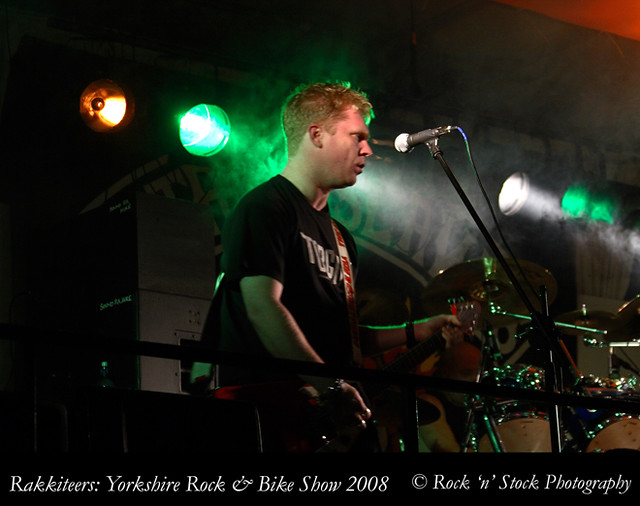The image captures a lively moment from the Racketeers performance at the Yorkshire Rock and Bike Show in 2008. On stage, a white male guitarist, aged around 35 to 40, with short blonde hair, is rocking out in a black T-shirt with white lettering. He holds an electric guitar, its strap slung over his shoulder, and stands in front of a microphone, hinting at his dual role as a singer. The stage is bathed in dynamic lighting, featuring green, yellow, and white spotlights, alongside atmospheric smoke from a smoke machine, creating a vibrant ambiance. To the right, a drum kit is visible, its cymbals reflecting the stage lights. At the bottom of the image, a black border displays the white text, "Racketeers Yorkshire Rock and Bike Show 2008. © Rock and Stock Photography," providing context and date for the event. The entire scene evokes the energetic spirit of a small, electrifying live music venue.